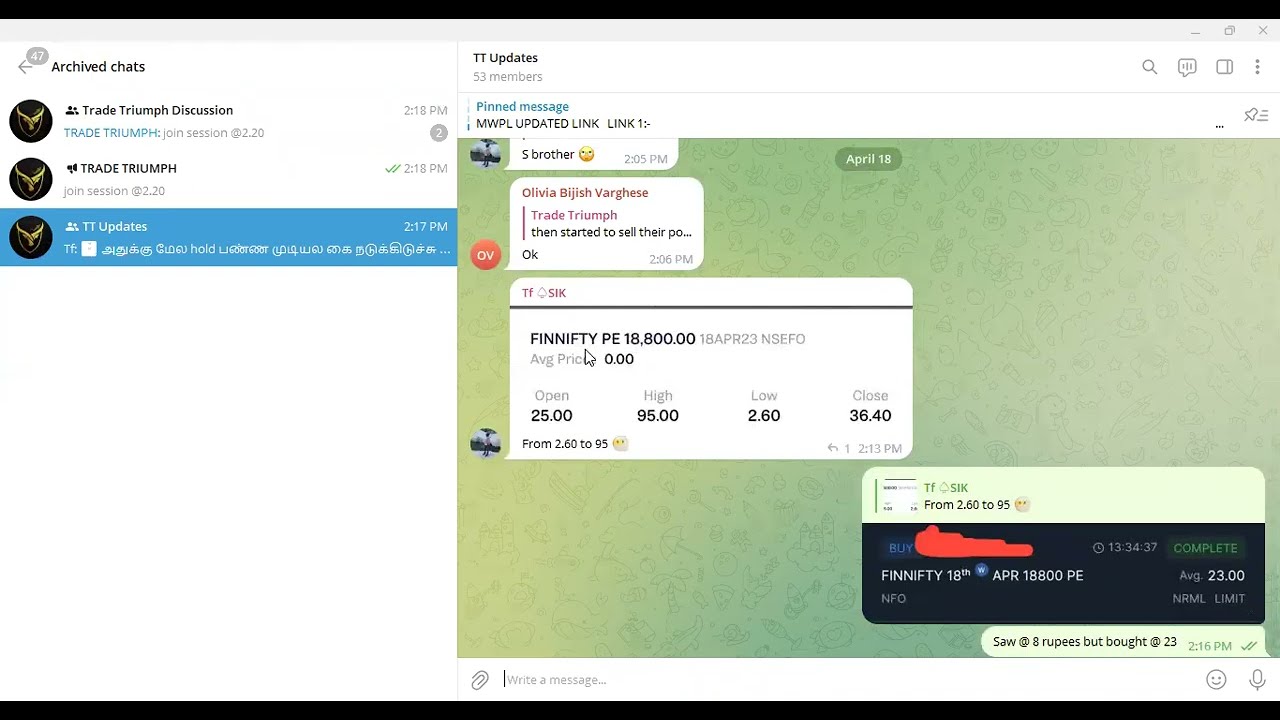The image is a computer-generated screenshot of a website featuring a chat interface. On the left-hand side, there is a section labeled "Archived Chats" with three entries: "Trade Triumph Discussion," "Trade Triumph," and "TT Updates," with "TT Updates" currently selected. The TT Updates chatroom includes 53 members and features a pinned message with an updated link. The background of the chat interface is green. Within the chatroom, there is an ongoing conversation between participants identified as S brother and T-sock. They appear to be discussing stock market transactions, mentioning prices such as "open 25," "high 95," "low 260," and "close 3640." A specific detail noted is S brother mentioning selling at "eight rupees but bought at 23." Also, the chat is dated April 18, though the year is not specified. Finally, the website address is not visible in the screenshot.